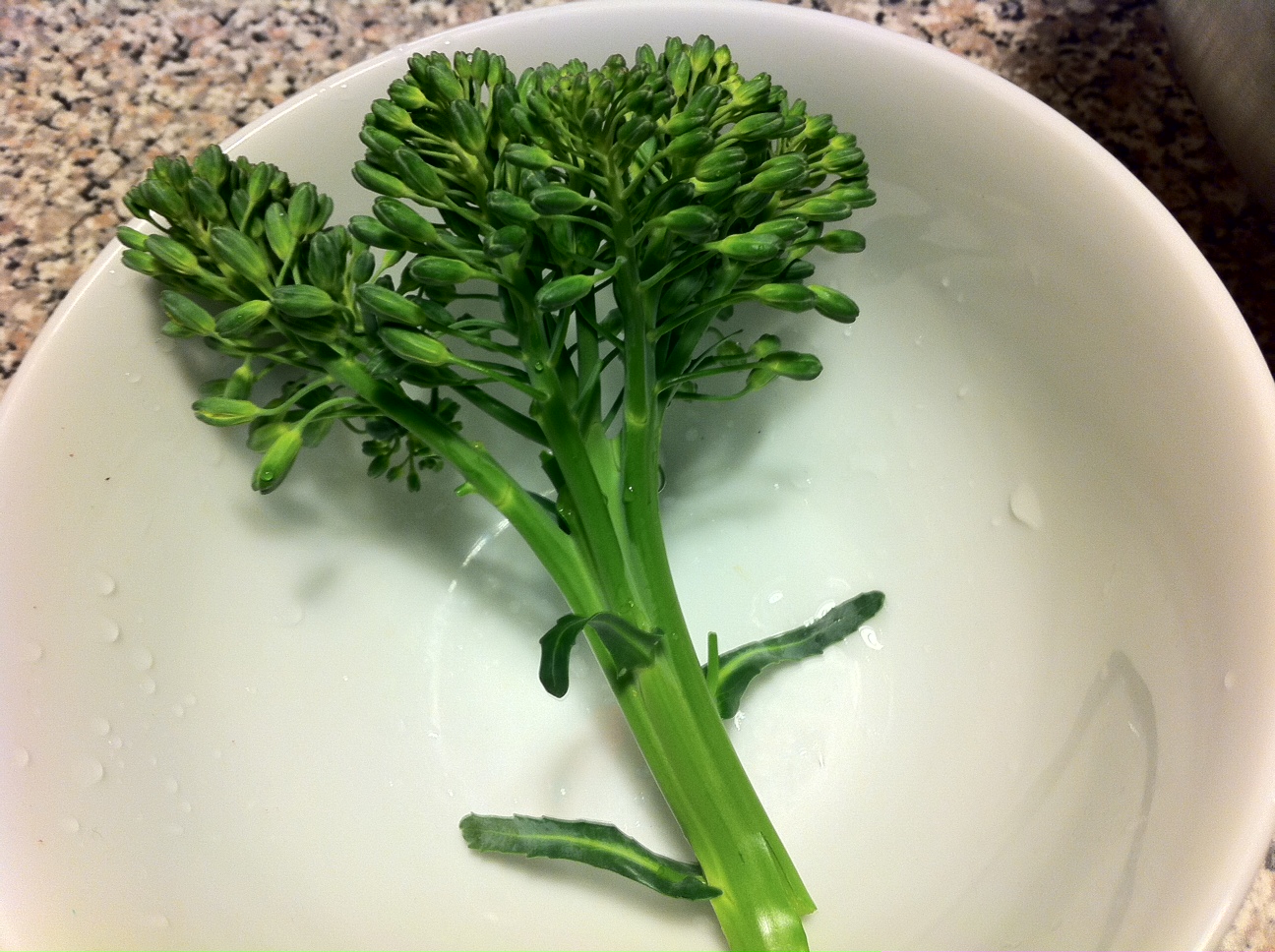This close-up, color photograph captures a piece of broccoli on a white plate set atop a granite countertop. The broccoli features a thick green stalk branching into three smaller stalks, each adorned with spindly green leaves and facing to the right, while the main stalk points left. Flecks of water on both the broccoli and plate suggest the vegetable has been recently washed. The granite countertop beneath the plate exhibits a sandy grain pattern, blending shades of tan, black, and white which is slightly blurred around the edges, contrasting against the clear, detailed focus on the broccoli and water droplets.